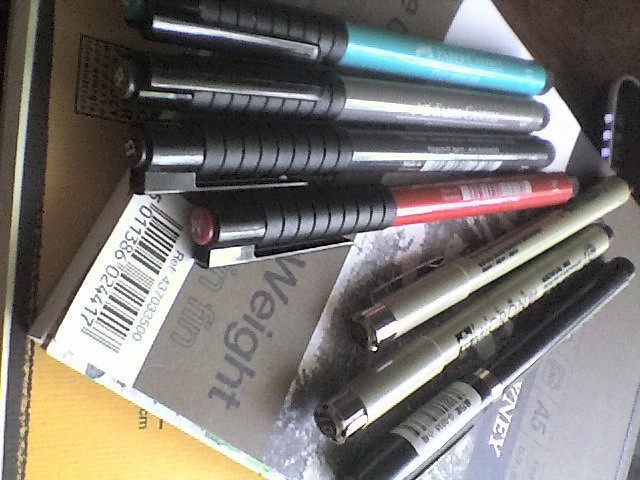In this image, an artist's sketch pad and a tablet with a closed cover are prominently displayed. Resting diagonally across the tablet are seven artist pens, each meticulously placed. Among them are three neutral-colored Pigma Micron ink pens, which are either black or very dark gray, known for their precision and reliability. Accompanying these are four Faber-Castell artist drawing pens, showcasing an array of colors: vibrant scarlet red, classic grey, sleek silver gray, and a soft light blue. This carefully arranged collection of tools hints at an artist ready to bring their creative visions to life.